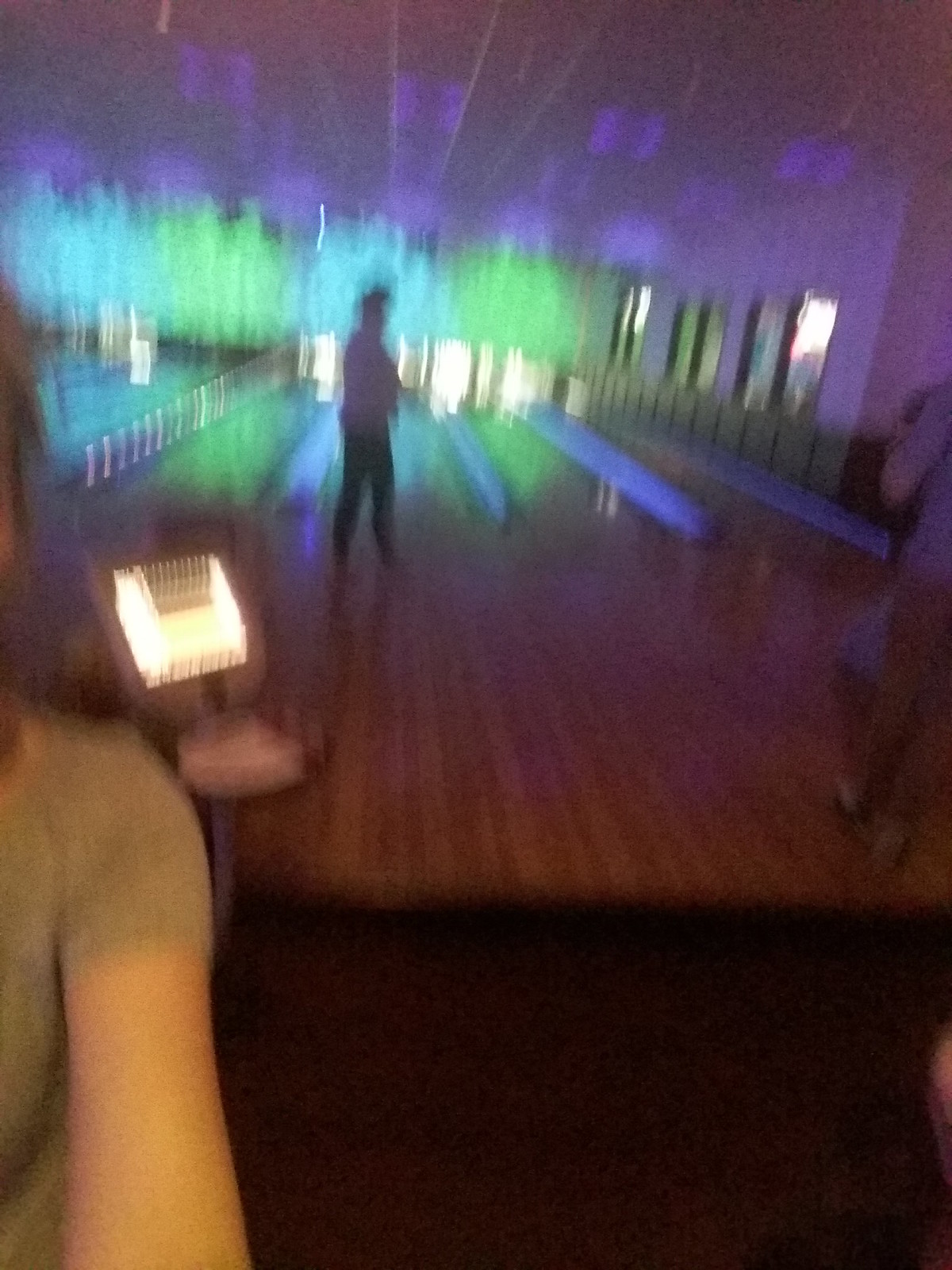This image depicts an extremely blurry interior of a bowling alley, captured from a woman's perspective at a bar. On the left of the image, partially visible is the woman herself, with long, brown hair draped over her shoulder, wearing a brownish-gray shirt. Her arm extends off-screen as she holds her phone towards the lanes behind her. The foreground features dark brown, textured wood floors. 

Centrally, the lanes typical of a bowling alley are visible, separated by gray cylindrical dividers. Standing in front of one of the lanes is a person, with a wide stance, dressed in black pants and a purplish shirt, appearing ready to bowl. In the background, multiple, blurred green and blue lights shine above the lanes, adding to the image's indistinct quality. To the right, another figure can be noticed, wearing brown pants, partially cut off by the frame. The back of the alley shows a lit-up screen, windows, or possibly posters hanging on a wall, further shrouded in the photo's overall blur.